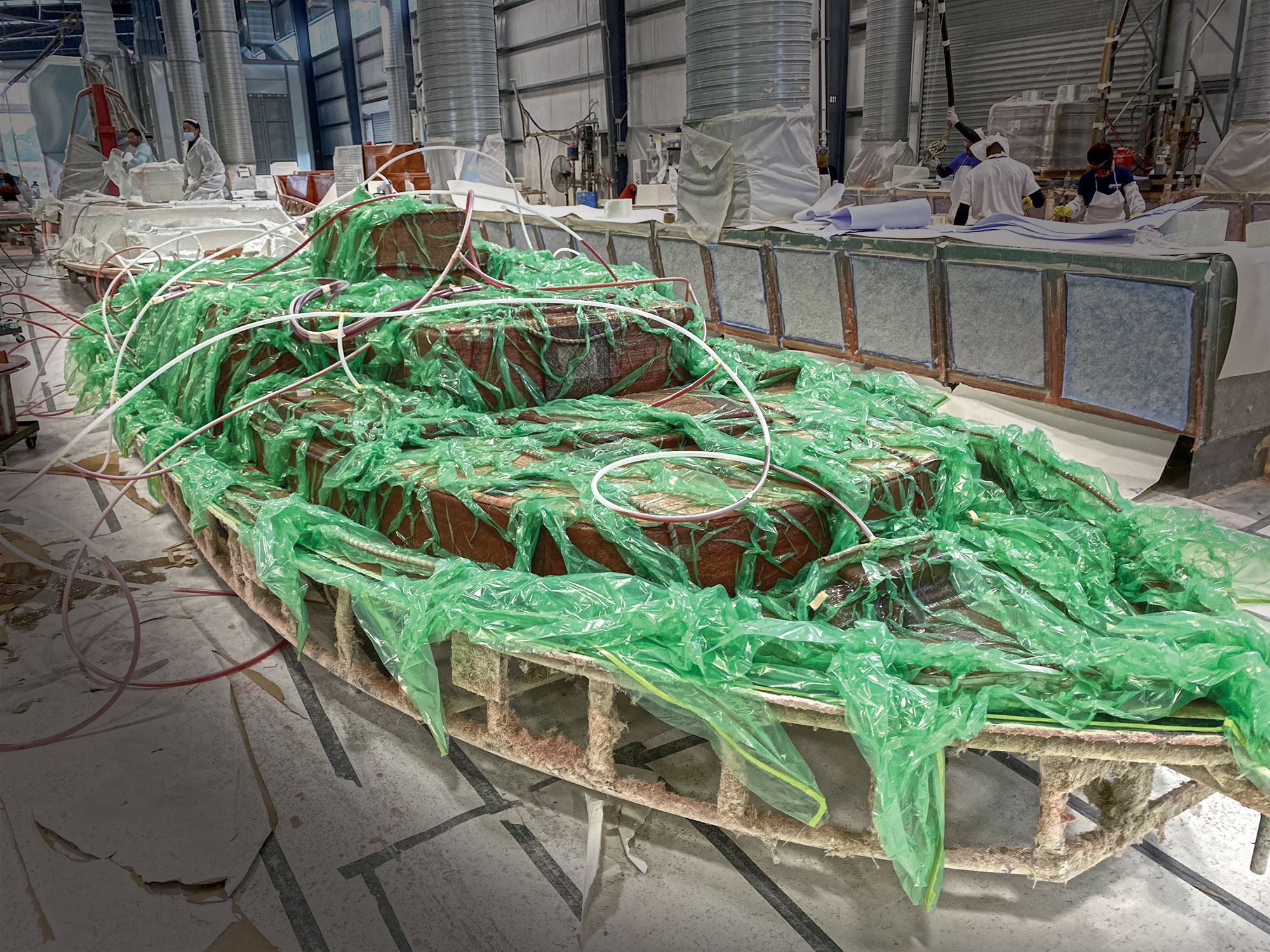In a sprawling, sterile warehouse resembling a boat-building factory, a massive, partly-constructed ship dominates the gray paper-covered ground. The boat, visibly aged with a rusted light brown metal frame at its base, is shrouded in a voluminous green plastic tarp, reminiscent of moss, enveloping the vessel from bow to stern. Emerging from this tangle of plastic, the darker-brown wooden structure of the boat, adorned with two levels of wooden platforms, stands out prominently.

At the very bottom of the boat's metal frame, light brown and rusted bumper-like sections connected by vertical bars can be seen, all marred with dust, dirt, and growths. Running along the top of the ship is a large rope, integrated into the vessel’s framework. 

The ship is oriented towards the right side of the photograph, where pairs of red and white piles can be seen atop it. In the background, figures clad in white uniforms and medical masks can be observed working near countertop areas. These workers, possibly scientists, add a clinical feel to the warehouse with its clean, white garage doors and long tubular structures reaching towards the ceiling. The scene hints at meticulous, ongoing work on the ship amidst an environment where other white boat-like objects and equipment are scattered, suggesting a bustling yet orderly industrial atmosphere.